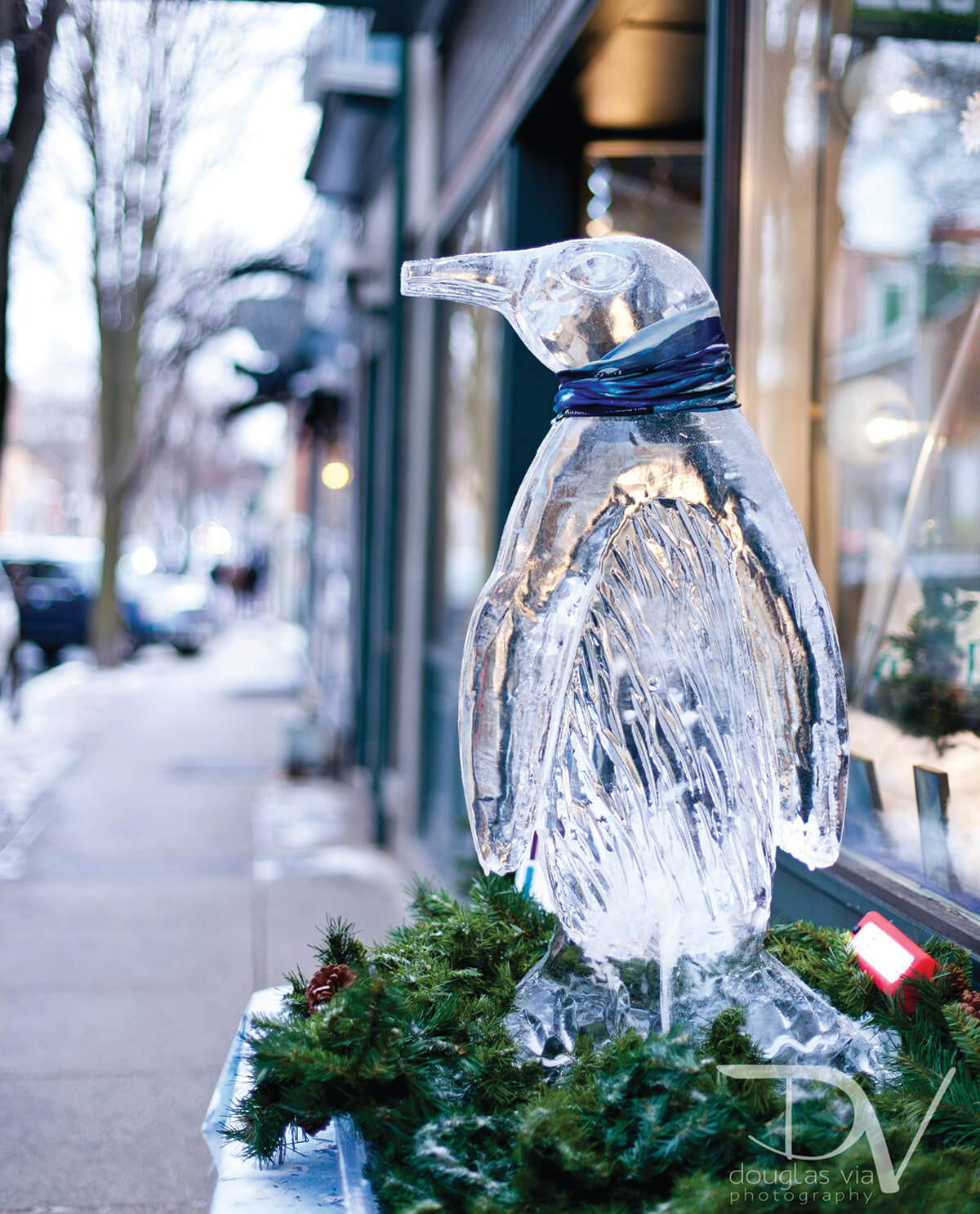The photograph captures a quaint storefront on a city sidewalk during a cold, winter day. Prominently displayed in front of the store is an intricately crafted glass sculpture of a penguin, about a foot and a half tall, adorned with a small blue scarf. The penguin faces left while perched on a bed of spruce tree branches, dotted with a few pine cones, creating a festive display. The surrounding area shows signs of winter, with a light dusting of snow on the partially shoveled sidewalk and leafless trees in the distance. To the left is a blurred, black car parked along the sidewalk, while the background features dark, almost black storefront buildings with windows that provide minimal visibility into the interiors. A small red tag or display is visible to the right of the penguin. In the bottom-right corner of the photo, the credit reads "D.V. Douglas via photography," marking the photographer's acknowledgment.